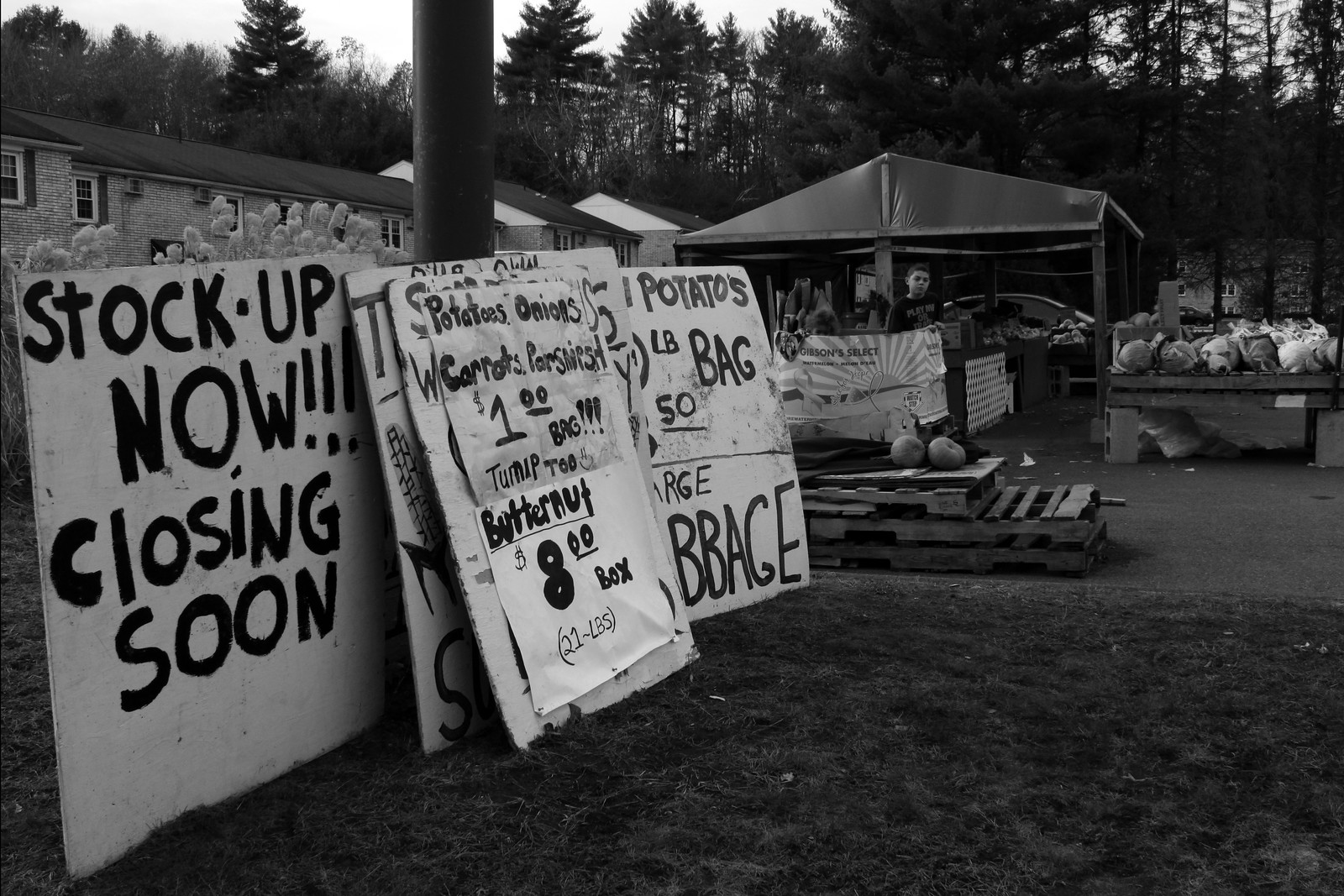In this black-and-white photograph, a scene from an outdoor farmer's market is captured, possibly as the day is winding down. In the foreground, a group of large, painted signs, prominently featuring messages such as "Stock up now, closing soon" and various produce prices—potatoes, onions, carrots, and parsnips for $1 a bag, turnips to butternut squash for $8 a box—are stacked and leaning against a pole. The signs are in white with black lettering, and some mention specific quantities like "21 pounds." Behind these signs, a few scattered pumpkins rest on wooden pallets, hinting at earlier bustling activity. Further back, tents or shelters with dark-colored cloth tops house the market stalls, possibly where transactions once took place. A counter, potentially for a cash register, is visible under one of the stalls. In the distant background, a couple of apartment buildings and some bushes are visible, setting a residential tone to the scene. The composition suggests it is probably evening as vendors appear to be packing up for the day.